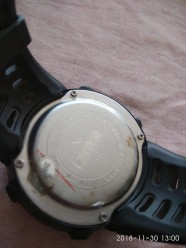The image features the back of a wristwatch prominently displayed. The view showcases the case back and the bezel, each fastened securely by four screws positioned at the corners. The watch is equipped with a black rubber strap, designed with vent holes for breathability. The timepiece rests on what appears to be a wrinkled white table cloth, adding texture to the setting. Notably, the case back of the watch displays a red streak of paint, likely from a recent scuff against a red-colored surface. Additional signs of wear and tear are visible, hinting at the watch's regular use.